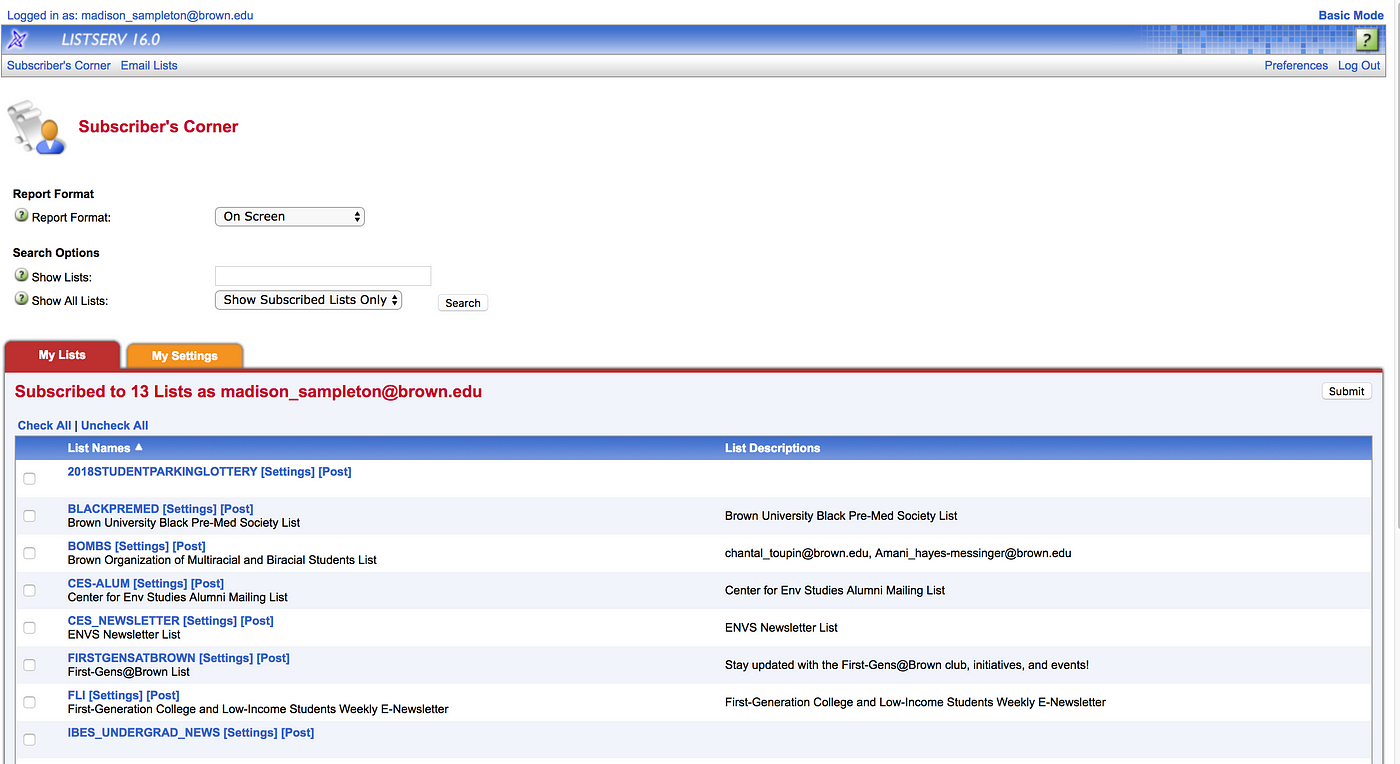The image depicts a computer screen displaying the interface of Listserv 16.0, showing it is accessed by Madison Sampleton from the domain trown.edu. The user is currently in the "Subscribers Corner" section, which presents a report format and various search options. In the report format, the search bar contains the term "on screen." Under the search options, there is a filter set to "show subscribed lists only." Below these search tools, two tabs are visible: the "My Lists" tab in red and the "My Settings" tab in orange.

Further down, there is a statement indicating that Madison Sampleton is subscribed to 13 lists as madisonsampleton@brown.edu. A list of names, displayed in blue, outlines the subscribed lists. The names of the lists include:

1. 2018 Student Parking Lottery
2. Black Pre-Med
3. BOMBS
4. CES Alum
5. CES Newsletter
6. First Gen at Brown
7. FLJ
8. IBS Undergrad News

The screen provides a detailed view of Madison Sampleton's Listserv subscriptions and their navigation options within the interface.